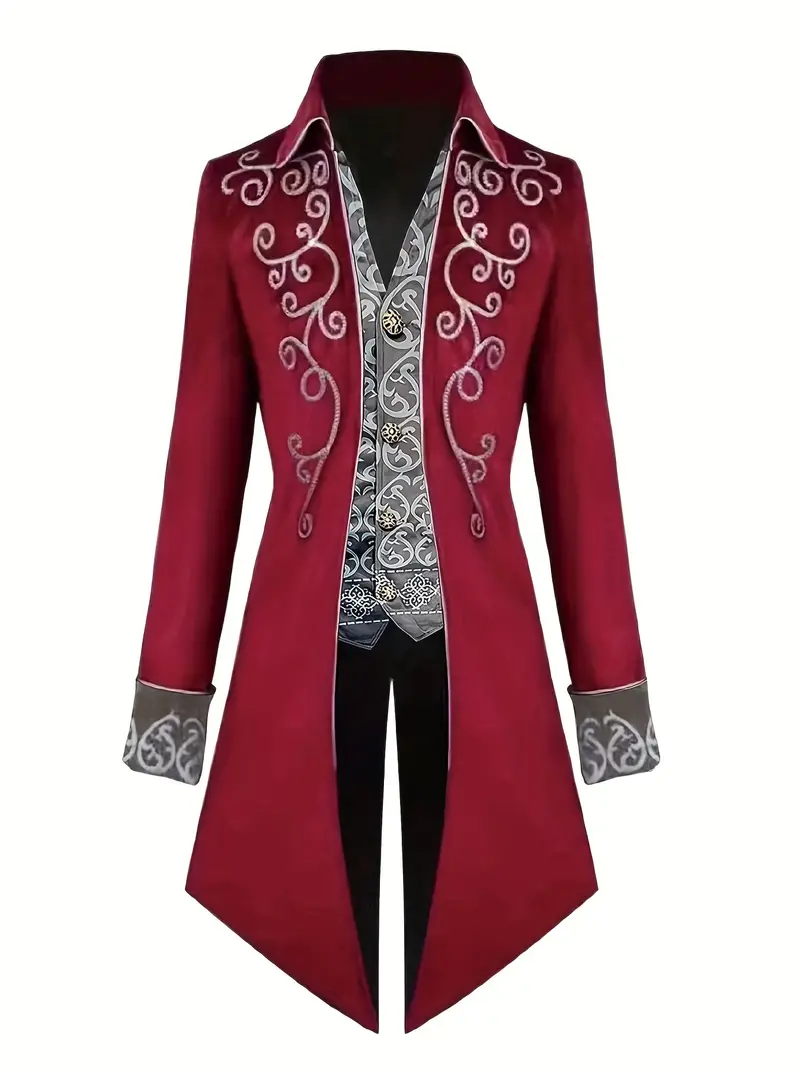The image depicts an elegant and formal outfit resembling a historic or royal attire displayed against a plain white background, which gives the impression that the garments might be floating in space. The centerpiece is a gray vest adorned with intricate white curly patterns, featuring three prominent decorative silver buttons arranged vertically from top to bottom. The vest assumes a V shape and appears to be positioned centrally in the image.

Encasing the vest is a long, regal red coat, which starts broad at the shoulders, narrows at the waist, and flares out slightly to form sharp diagonal points at the bottom, almost like an hourglass figure. The coat has a black interior trim visible along its insides and coat tails that come to pointed ends. The coat also includes elaborate white embroidery running from the collar down to the lapels, mimicking a design found on historical garments. This embroidery extends to the gray cuffs, enhancing the formality of the outfit.

Above the coat, a collar extends outward, framing the top of the ensemble. The entire attire, devoid of any buttons or zippers on the coat itself, suggests an open, flowing design suitable for an upscale presentation or a prestigious event from the 19th century. It appears to be displayed on a black mannequin, emphasizing its formal and majestic nature.